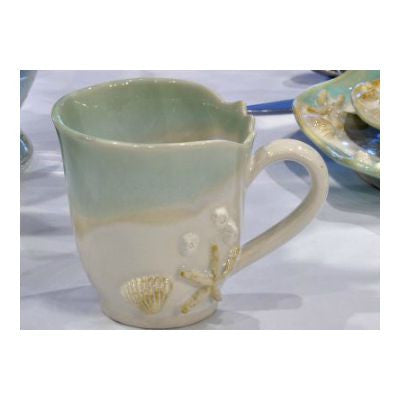This image showcases a detailed ceramic coffee mug designed with a vibrant beach theme. The bottom of the mug features intricate seashell and starfish patterns, which are golden and white in color, designed to resemble a sandy beach. The base of the mug transitions from a light beige into a wavy-edged opening, adorned in a soft, glazed teal that fades into a greenish turquoise hue near the lip. The overall design gives a sense of tranquility and coastal charm. The mug, with a handle that matches its ceramic build, sits gracefully on a dinner plate which carries the same seashell and starfish patterns. A silver butter knife is placed next to it. This entire setup rests elegantly on a white tablecloth, adding a touch of simplicity and contrast to the detailed and colorful beach-themed ceramics. In the background, faint blue hues provide a serene backdrop that complements the seaside aesthetic of the mug.